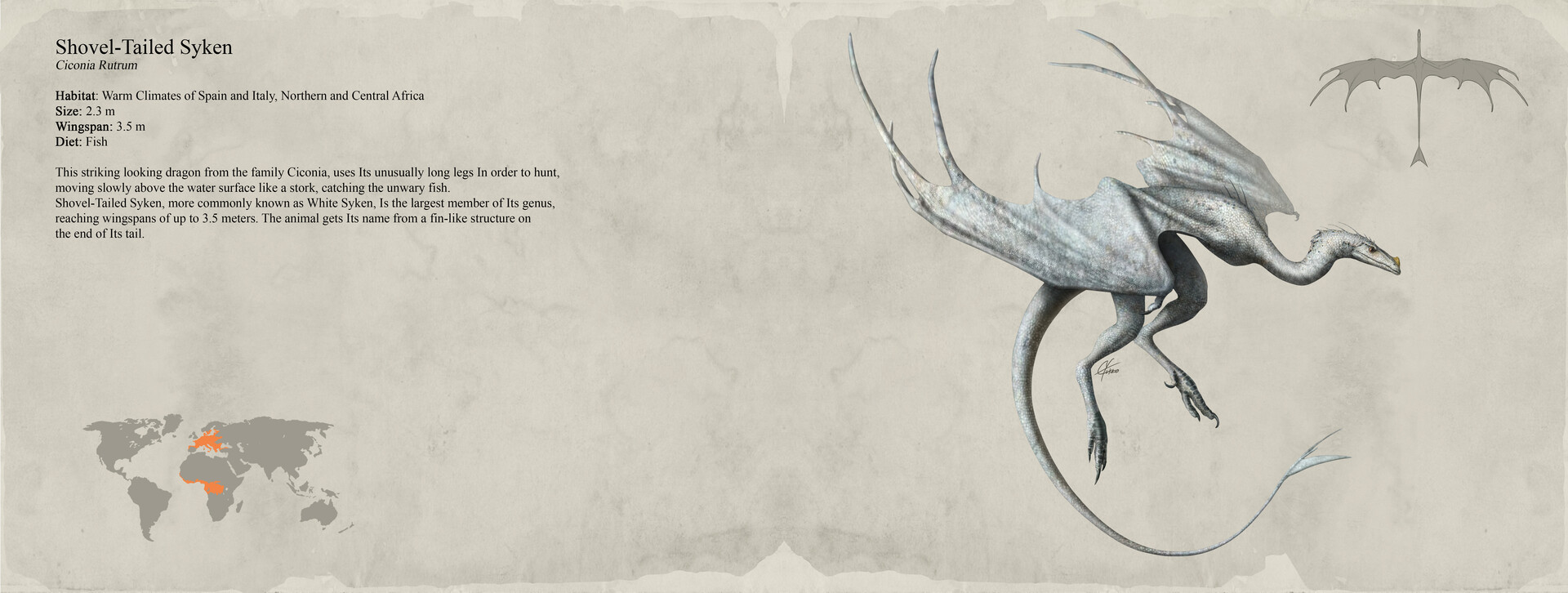This detailed image resembles a textbook entry documenting a mythical dragon, identified as the Shovel-Tailed Saikhan. Featuring a compelling depiction, the dragon has two large wings, a dragon-like head, a long, fin-ended tail, and two elongated legs which it utilizes for hunting. The creature's wingspan, noted to be 3.5 meters, and its overall size of 2.3 meters are meticulously illustrated, with an aerial view displaying its impressive wingspan. The texture of the image mimics aged, torn papyrus, enhancing its antique appearance.

The Shovel-Tailed Saikhan is predominantly found in the warm climates of Spain, Italy, and stretches across northern and central Africa, with these regions highlighted on a map located in the bottom left corner. Its diet consists primarily of fish, which it captures by moving slowly above the water's surface using its long legs, similar to a stork's hunting technique. The name 'Shovel-Tailed' derives from the fin-like structure at the end of its tail. Despite its striking silver-white appearance and considerable size, the dragon is described as not overly menacing. Additional notes mention it as the largest member of the Ceionia family, emphasizing its distinct characteristics and ecological niche.